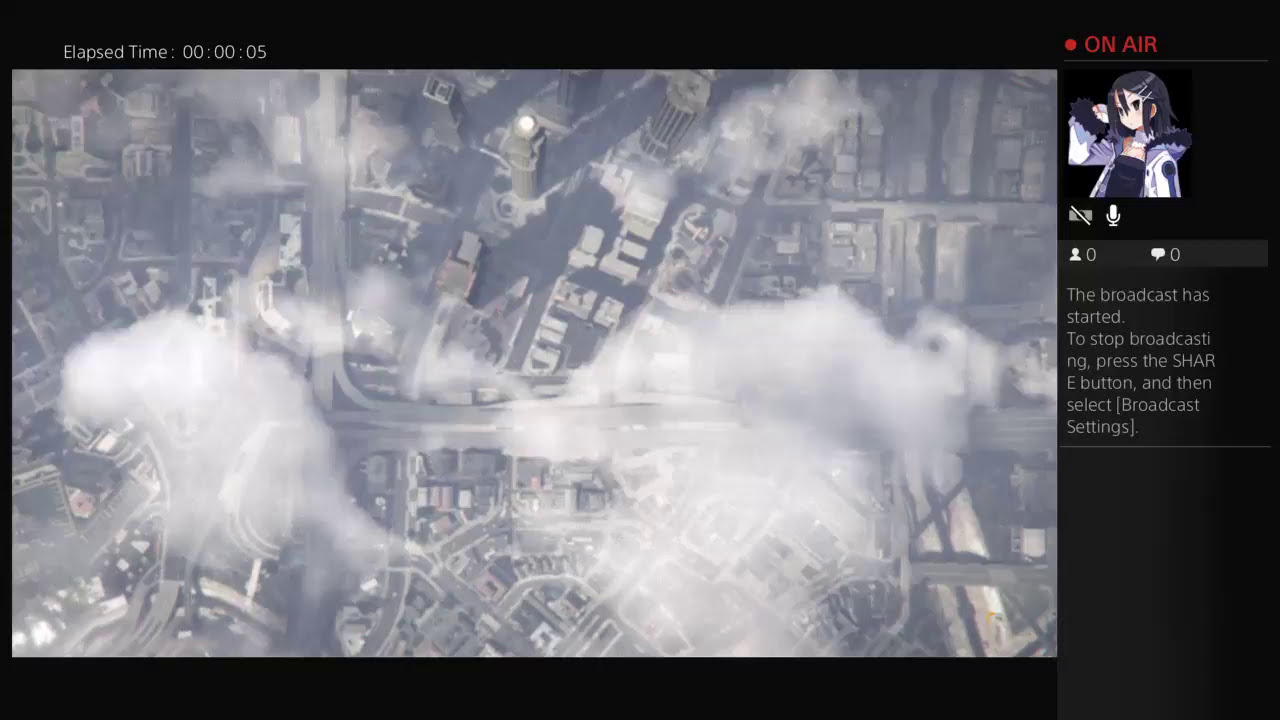This screenshot appears to be from a PlayStation 4 streaming interface, capturing a live broadcast of what seems to be a video game, possibly resembling the bird's-eye view style of Grand Theft Auto. The main section of the image is a black-and-white photograph positioned towards the left edge, depicting the chaotic scene of a building mid-destruction with twisted metal, tilted structures, and rising smoke from piles of debris. The background is predominantly black, accentuating the dramatic visuals.

On the right-hand side of the image, there is a series of elements embedded within the black background. At the top, red text with a white dot reads "on air," indicating the live stream status. Below this, a square displays an anime avatar or character. Further down, a crossed-out symbol followed by a white microphone icon is visible, likely part of the streaming interface features. 

The interface also includes two columns, each marked with the numeral zero, probably indicating the number of spectators and comments, with some unreadable white text below them. At the top of the image, the elapsed streaming time is shown as "00:00:05." The black border at the top includes additional text providing instructions: "The broadcast has started. To stop broadcasting, press the share button and then select broadcast settings." The overall hazy, bluish tone implies a significant aerial distance, viewing what appear to be residential areas and skyscrapers partially obscured by clouds, adding to the intricate detail of this dynamic screenshot.